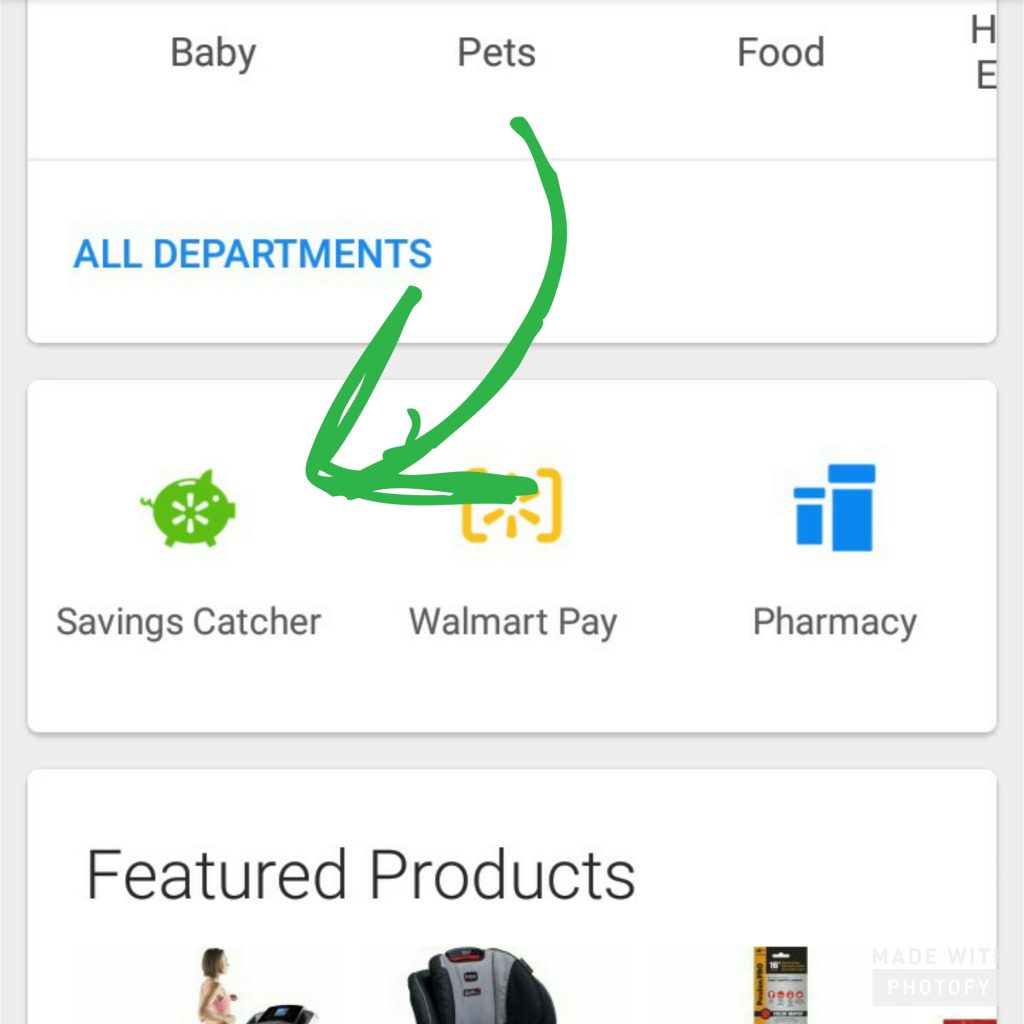A cropped screenshot of a Walmart website or app interface is displayed. At the very top, several departmental categories are visible, including "Baby," "Pets," "Food," and another section starting with an "H" that is cut off. Below these categories is an "All Departments" section. A green arrow has been annotated or drawn onto the image, pointing to an icon under the "All Departments" section. 

The subsequent section contains options labeled "Savings Catcher," "Walmart Pay," and "Pharmacy." The green annotated arrow specifically points to the "Savings Catcher" option, which is represented by a green piggy bank icon featuring the Walmart symbol. Next to this, "Walmart Pay" is indicated with a yellow icon encased in brackets, displaying the Walmart symbol. The "Pharmacy" option is marked with a blue icon depicting pharmacy bottles.

Beneath this section, there is a partial view of the "Featured Products" area. The top edges of a woman exercising, a baby seat, and an item that appears to be a medicine or fertilizer can be glimpsed at the bottom of the cropped image.